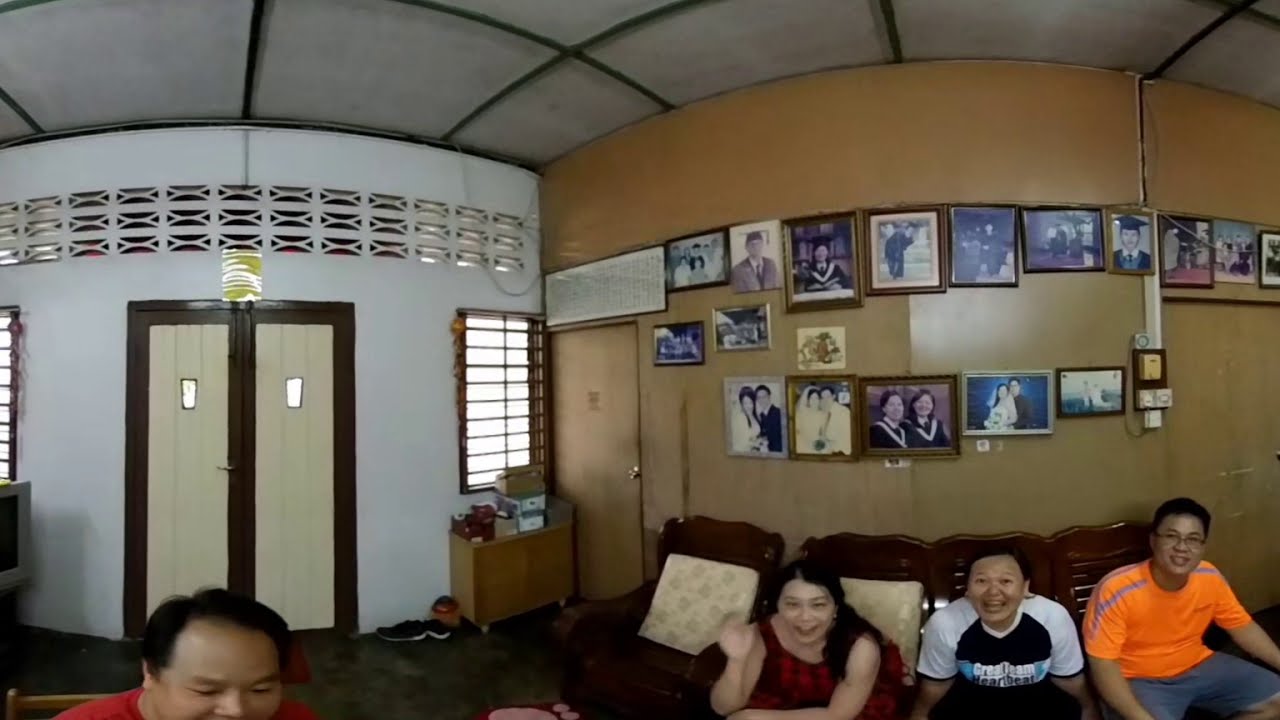This wide panoramic image captures a family gathering in a cozy, warmly-lit living room. Dominating the scene is a red three-seater sofa where two women and one man, all with Asian facial features, sit closely and smile directly at the camera. The woman on the left dons a red and checkered sleeveless dress, her long black hair cascading over her shoulders as she waves. In the middle, a middle-aged woman with black hair wears a t-shirt with white shoulders and short sleeves, featuring black and light blue stripes across the chest. To her right sits a clean-shaven man with short black hair and glasses, dressed in an orange t-shirt with gray stripes on the shoulders and blue shorts.

Behind the trio, a brown-colored wall is richly adorned with a plethora of framed photographs, showcasing family milestones such as weddings and graduations, adding a deeply personal touch to the space. In contrast, a white wall with rectangular cutouts for ventilation can be seen on the left, featuring a central dark brown double door with tan interiors. Near the left corner of the image, partially visible from the nose up, an older man with balding hair and wearing a red t-shirt is slightly leaned forward, looking downwards rather than at the camera.

Additional details include a beige-cushioned seat adjacent to the sofa, a nearby shoe cabinet with some shoes scattered around, and a visible gray ceiling. The left corner also reveals part of a television, hinting at the homely environment. This detailed composition of the scene conveys a sense of warmth and shared happiness amongst the family members, captured in a single, cherished moment.